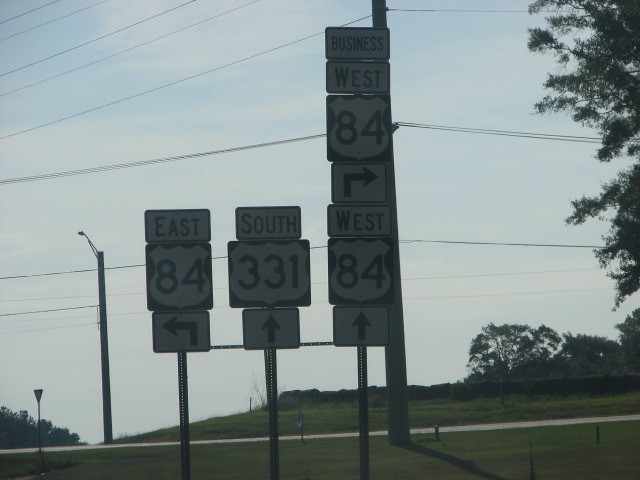This color photograph, taken on a somewhat cloudy and overcast day, captures a scene along the side of a road featuring multiple road signs and surrounding elements. From left to right, there are three signposts, each indicating different routes. On the far left, the top sign reads "East 84" with an interstate sign below it and an arrow pointing left. The middle signpost features a "South 331" sign with an accompanying arrow pointing straight. The signpost on the right is the tallest and most complex; at the top, it says "Business West 84" with an arrow pointing right, followed by another sign below it that states "West 84" with an arrow pointing straight. The background reveals a green field, trees, a few rolling hills, and a tall electrical pole with wires extending from various levels. The photograph also includes power lines scattered throughout and a railing at the bottom, as well as scattered trees and a triangular-shaped sign in the foreground. The overall lighting is dim, contributing to the slightly unclear quality of the image.